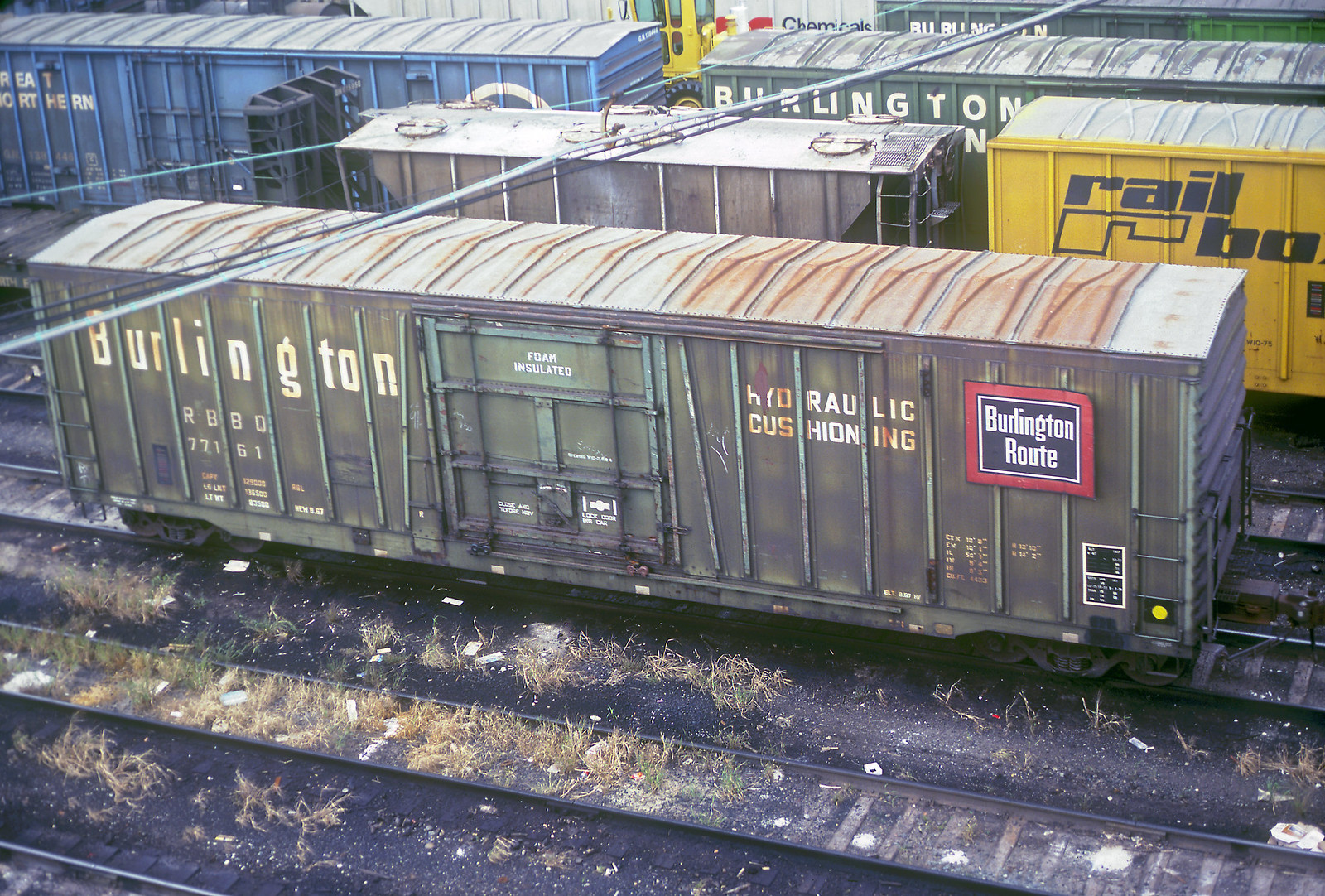The image showcases a weathered train yard with multiple rusted and faded freight cars lined up on overgrown railroad tracks. The focal point is a green Burlington freight car, centrally positioned and extensively weather-beaten, with notable rust streaks and a roof faded to a light gray. The sides are marred by prominent rust patches, and on the far left, faded white lettering reads "Burlington" with "RBBO" just below it, followed by the numbers "77161" and other smaller, unreadable text. The car features a door marked with "foam insulated," and towards the right, text indicating "hydraulic cushioning" amidst rust stains. A red square on the right displays "Burlington Route" with a black square beneath it containing white lettering. A ladder runs halfway up the right side, highlighted by a yellow dot at its base. Surrounding this car, the tracks are interspersed with weeds and grass, suggesting long-term disuse, further evidenced by broken wooden planks along the tracks. In the background, a succession of freight cars can be seen: a gray car, a yellow car to the right, a blue car, and another green Burlington car, all set against a backdrop of power lines, a building labeled "Chemicals," and what appears to be a yellow tractor. The overall scene conveys a sense of abandonment and decay, characteristic of a once-active freight yard now overtaken by time.